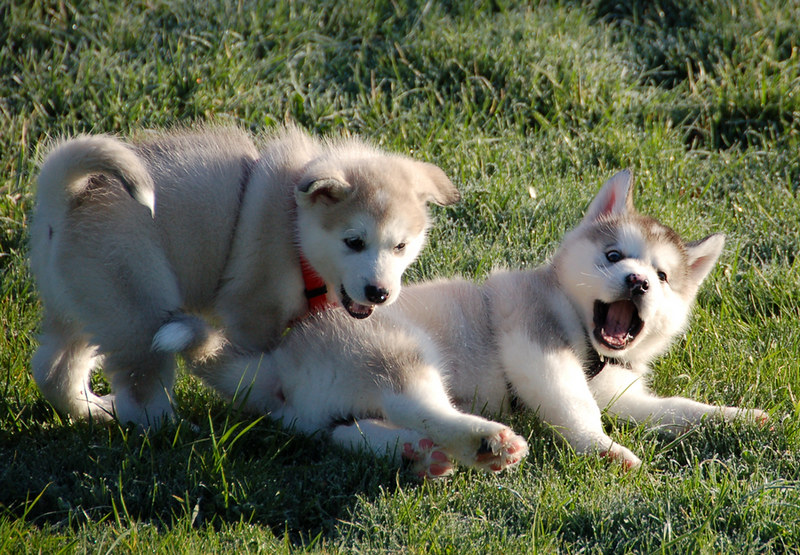This outdoor photograph captures an adorable and lively scene featuring two playful Siberian Husky puppies amidst a lush, green field of grass. In the center of the image, the puppy on the right is lying on its side with all four feet splayed to the right, its mouth open and eyes wide, giving a look of surprise. This puppy, with fur that is a mix of white and gray, wears a collar that appears to be black, although it's partially obscured by its position. Its ears are pointed and perked up, enhancing its shocked expression. To the left, another puppy, sporting a red collar, is energetically running towards and stepping on its sibling. This playful pup has curved, flappy ears, giving it a younger and sillier appearance in contrast to its surprised sibling. The puppies, exhibiting traits like pink paws, short tails with white tips, and tiny snouts, also have subtle variations in fur tones, with hints of brown on their heads. Shadows cast by the puppies can be seen on the grass, adding depth to the scene. Both puppies have short limbs and are fully immersed in their playful antics, making this a heartwarming snapshot of their joyful interactions.